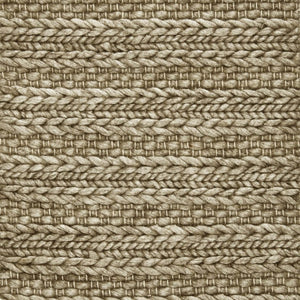The image showcases a highly detailed close-up of a rectangular piece of crocheting work in a light brown, taupe-colored material with subtle grayish and white highlights. The intricate pattern is arranged horizontally, starting from the top with small rectangular stitches. This is followed by a braided section that features arrow-like shapes pointing to the right, then a thinner braid with arrows pointing to the left. Another thicker braid follows with arrows pointing to the left, mirroring the top braid, before the rectangle pattern repeats. Overall, the image captures the texture and complexity of the crocheting stitches, highlighting varying thicknesses and detailed, alternating braid patterns.